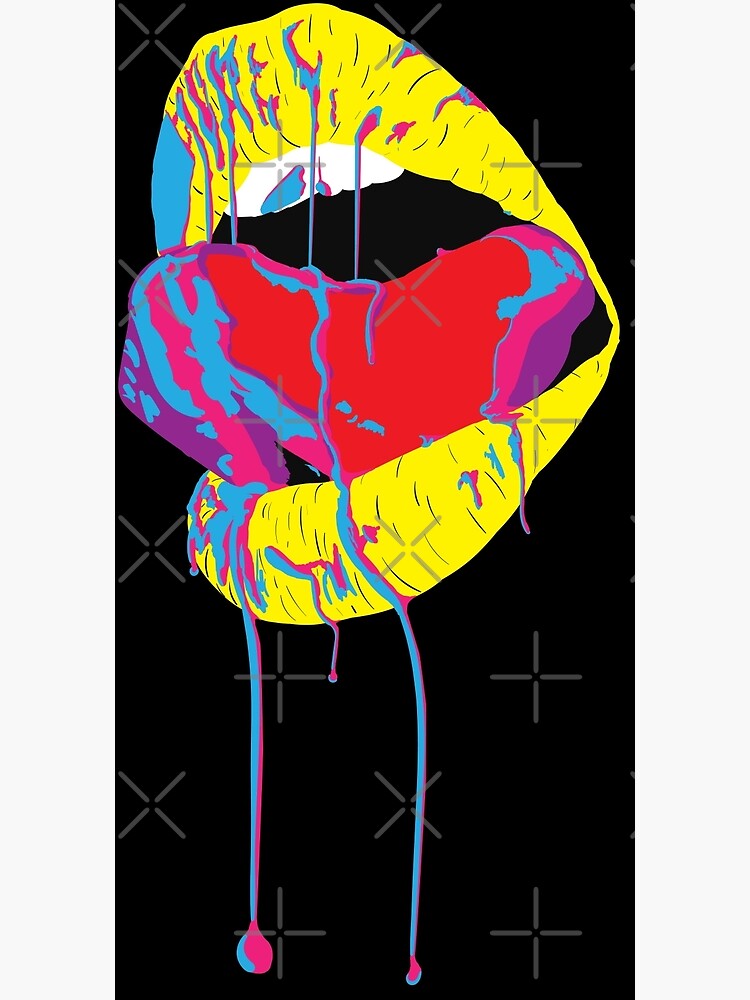This graphic painting, twice as tall as it is wide, showcases a striking pop art style image with prominent yellow lips against a solid black background. The mouth is angled at about 45 degrees towards the left side, revealing a red tongue sticking out suggestively and partially visible top teeth. The lips and tongue are adorned with dripping liquids in vibrant hot pink and medium blue hues, creating a dynamic visual effect. These drips cascade from the top lip, across the tongue, and down to the bottom lip, with some drops stretching further down. The background features translucent gray X's and plus signs as watermarks, subtly overlaying the dramatic, colorful scene reminiscent of the iconic Rolling Stones lips.